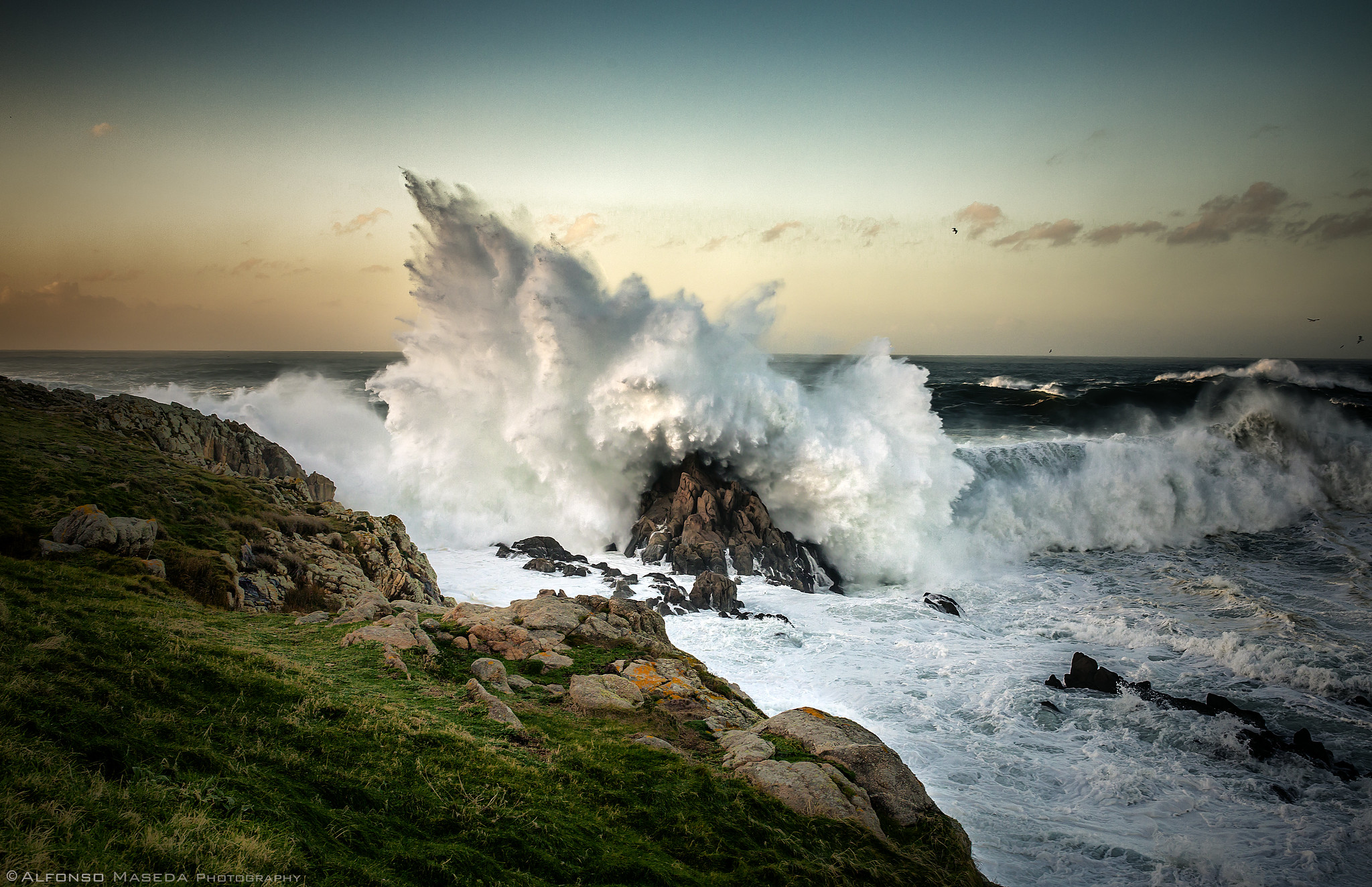In this captivating photograph, a powerful wave crashes dramatically against a towering, jagged rock formation just off the shore. The scene is set during the late hours of the day, with fluffy clouds lining the horizon and a subtle pinkish hue painted across the sky. The sun is hidden from view, possibly obscured by the massive wave, while the sky transitions to a deeper bluish tone as it stretches upwards. The photograph features some vignetting, which accentuates the gradient from the rosy horizon to the darker sky above. 

On the left side of the image, a grassy hill gives way to a rugged, craggy landscape that abruptly drops off into the tumultuous ocean, where the photographer stands. The rocky terrain is a light brown, contrasting with the near-black, almost dark brown, jagged rocks in the ocean, drenched by the relentless surf. The water is frothing with intense, white and green foam, creating intricate swirls and patterns in the turmoil. 

At the center of the composition, the wave crashes against the prominent rock, with the splash reaching astounding heights, likely at least 20 feet from the base of the rock to the crest of the splash. In the distance, another massive wave begins to break, hinting at the relentless power of the sea. The overall scene captures the raw, untamed beauty of the ocean at dusk, with its dynamic interplay of light, color, and texture.